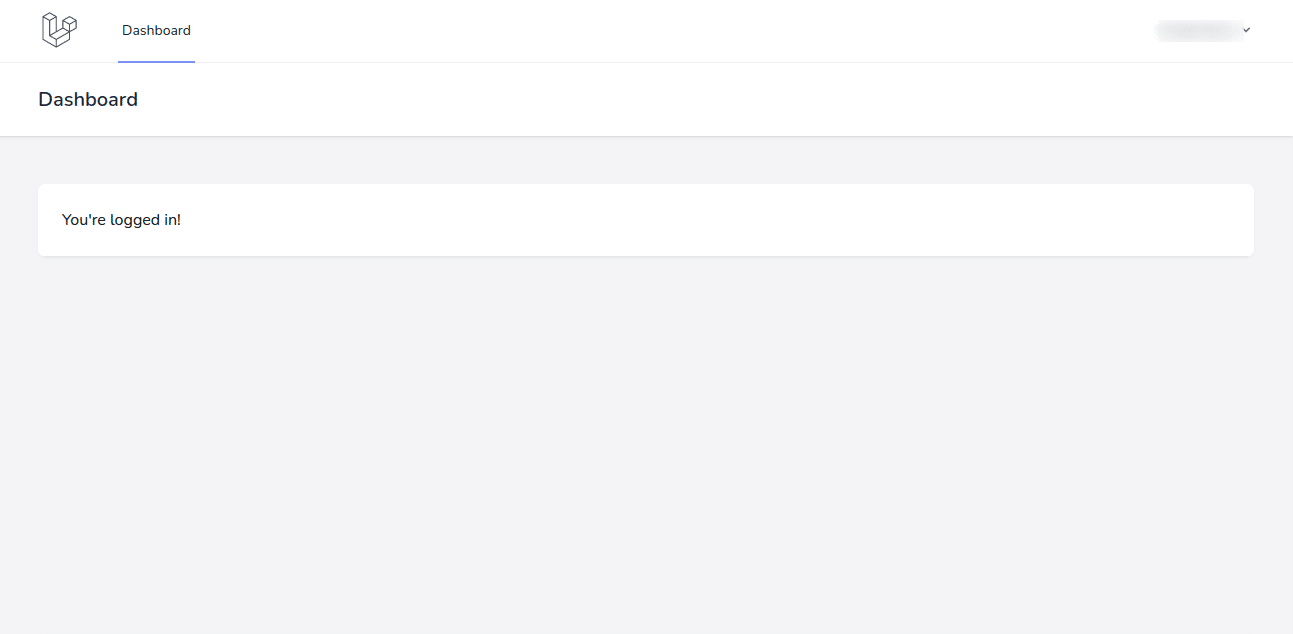A minimalist screenshot showcasing a user interface predominantly consisting of white and light gray colors. The top section of the page is white, transitioning to a light gray background below. In the upper left corner, there is a 3D stylized letter "L" icon accompanied by a smaller cube. To the right of the icon, the word "Dashboard" is prominently displayed with a blue line beneath it. Directly under the blue line, the word "Dashboard" is repeated. 

The main content area, set against the light gray backdrop, features a thin white box with the text "You're logged in." At the very upper left corner, there's a grayed out text indicating the presence of a potential drop-down menu, although no company name, customer details, or additional context is provided, leaving the purpose of the dashboard ambiguous.